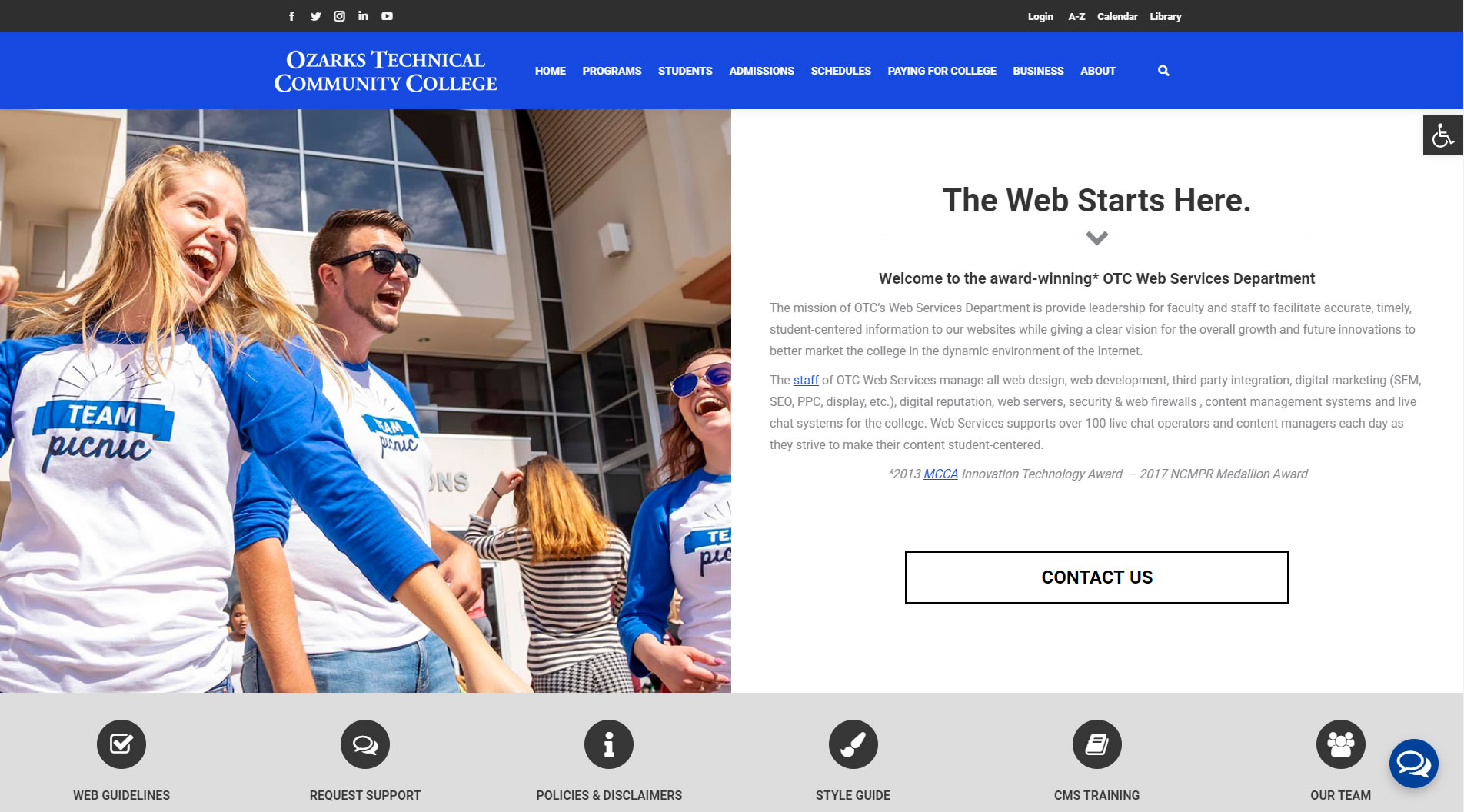In this lively and sun-drenched scene, a group of predominantly Caucasian individuals is captured enjoying a sunny day outside of a modern building with large, glass-like windows. At the center of the image, a blonde woman stands out in the sunlight, accompanied by a bearded man who is wearing glasses. To their right, two more women appear, one facing forward and the other with her back turned. These individuals are dressed in white shirts featuring blue sleeves, branding the phrase "Team Picnic," signifying a casual and communal event.

Behind them, the building's facade prominently displays a welcoming message, which reads, "The Web Starts Here." Below this header, the sign continues with, "Welcome to the Award Winning OTC Web Service Department," followed by "Contact Us." Additionally, the signage includes a variety of helpful widgets labeled Web Guidelines, Request Support, Policies and Disclaimers, Style Guide, CMS Training, and Our Team.

In the lower-right corner of the image, a chat bubble icon suggests the option to initiate a conversation with a representative, offering further assistance and information regarding the department. The overall setting exudes a sense of community and professional camaraderie, anchored by the inviting and informative backdrop.